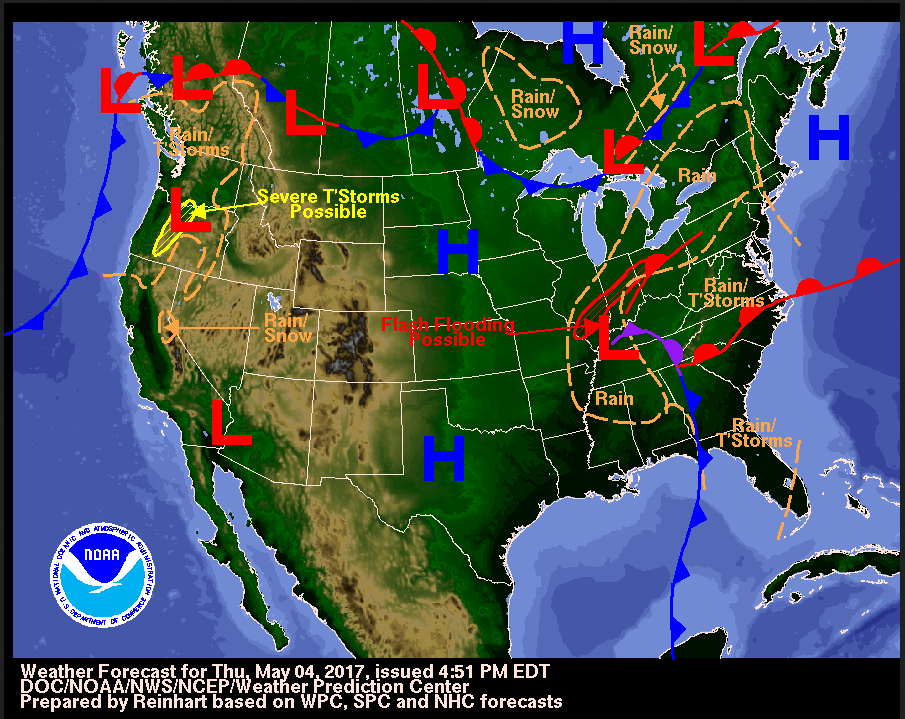This detailed weather map from the National Oceanic and Atmospheric Administration (NOAA), issued on Thursday, May 4, 2017, at 4:51 p.m. EDT, provides a comprehensive forecast prepared by Reinhart based on WPC, SPC, and NHC forecasts. The color-coded map highlights various weather conditions across North America, including the United States, Canada, Mexico, the oceans, the Great Lakes, and even Hudson's Bay. Prominent high-pressure zones are marked with blue H's, and low-pressure zones with red L's.

On the West Coast, especially around California and central Oregon, severe thunderstorms are anticipated with rain and snow in the lower regions. The central United States is at risk of flash flooding, particularly across southern Illinois, Indiana, and into Ohio. Rain and thunderstorms are projected throughout the Pacific Northwest and moving through the Ohio Valley down the Mississippi Valley. The Canadian border regions are predicted to experience rain and snow, particularly around Ontario and the eastern provinces.

Eastern U.S. states, from Florida up through Kentucky, will also face rain and thunderstorms. The detailed map also includes key geographical markers like the Great Salt Lake and the Everglades, and it features clear visual indicators such as blue and red arrows signifying various weather patterns.

The map's bottom-left corner displays the NOAA emblem, aligning with the overall highly organized presentation that uses a vibrant color scheme of red, blue, yellow, and green to clearly denote different weather conditions. This visually appealing and informative map encapsulates a broad range of meteorological phenomena, providing a vivid and accessible forecast for all regions covered.